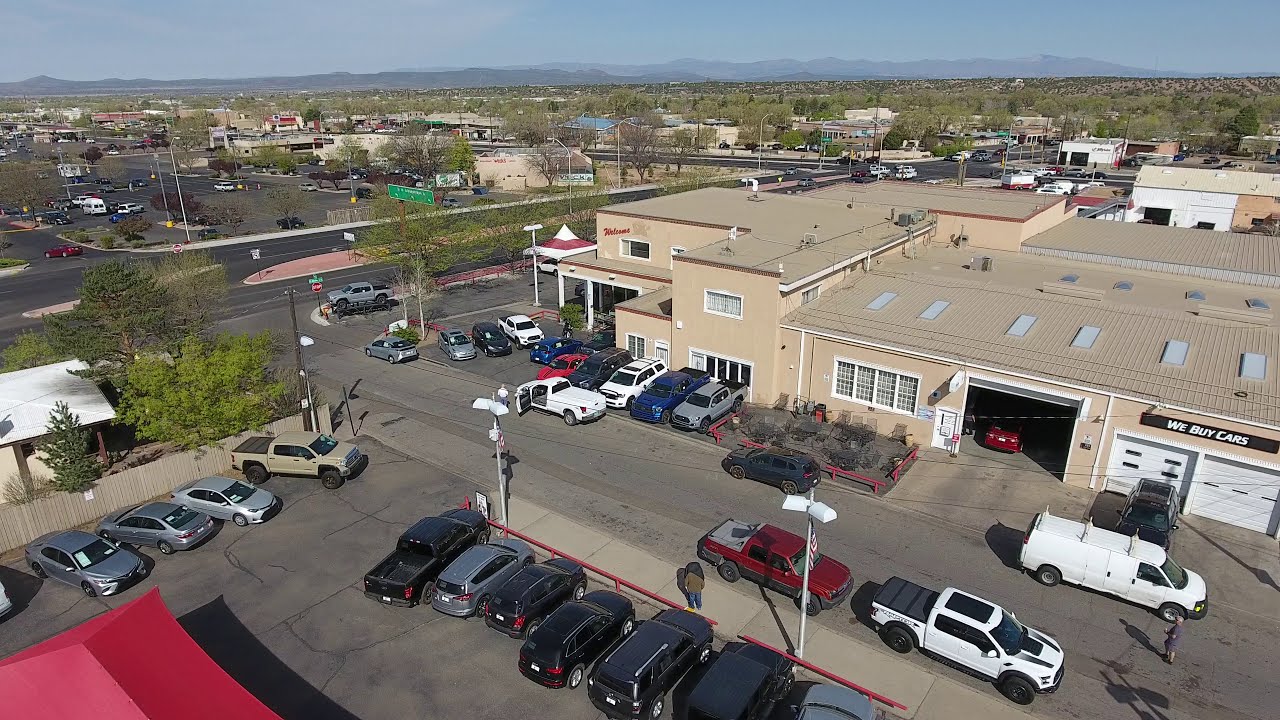In this detailed aerial photograph, we see a sizable tan building with white trim and a flat, grayish roof equipped with solar panels. A bold sign declaring "We Buy Cars" is prominently displayed on its facade. The building features several white and gray windows and includes both closed and open white garage doors. A black car is parked by one of the closed garage doors, while a red car occupies the open one. 

In front of the building, there’s a red brick garden, bordered by a cluster of trucks. This area is set alongside a gray street, identified as Tulane Road, which has a distinctive red median. Across the street from this building, another lot boasts numerous cars for sale. Also noticeable in the vicinity is a green highway sign, though its text remains unreadable.

Surrounding the area, other commercial and industrial buildings are visible, all set against a backdrop of heavily tree-lined surroundings. In the distance, a light brown mountain range rises under an overcast, bluish-gray sky, adding a natural frame to the urban scene.